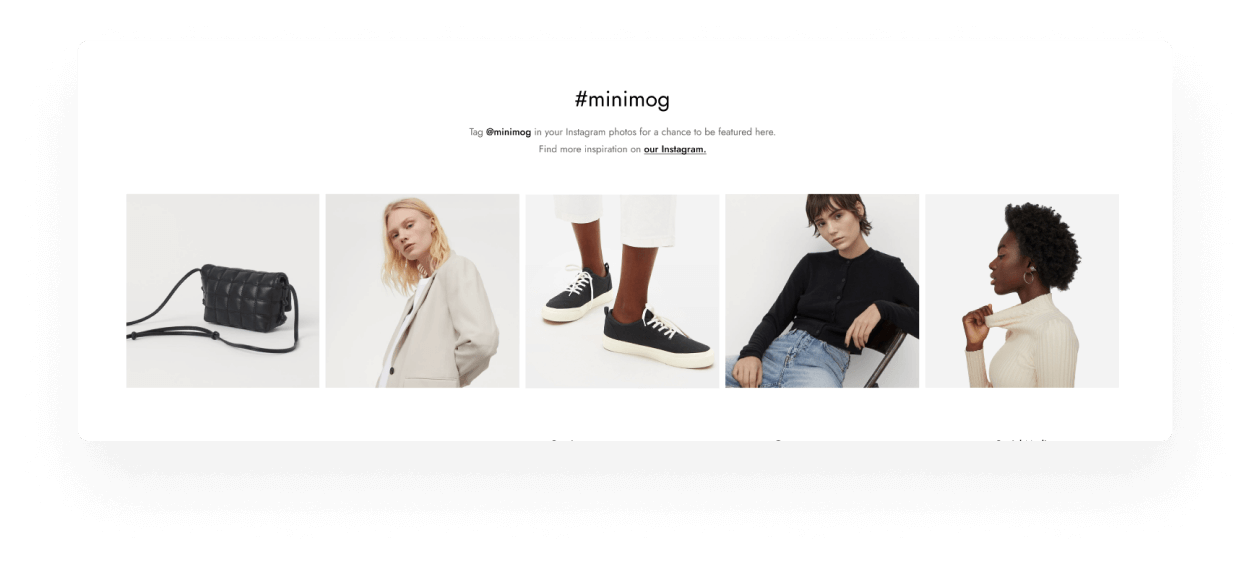A detailed screenshot captured from a laptop displays a social media prompt from the brand Minimog, set against a white background. At the top of the image, bold black lettering features the hashtag "Minimog" (hashtag #MINIMOG). Below this, the text encourages followers to tag their Instagram photos with @Minimog for a chance to be featured. The instruction reads, "Tag @Minimog in your Instagram photos for a chance to be featured here." 

Following this, the message urges viewers to find more inspiration by exploring their Instagram profile, indicated by the text "Find more inspiration on our Instagram," with "our Instagram" underlined and bolded, resembling a hyperlink.

Beneath the textual content, the image showcases a row of five customer-tagged photos displaying various products associated with the brand. From left to right, the images include a sleek black handbag, a young blonde woman gazing directly into the camera while wearing a white jacket, a pair of elegant black shoes, a woman wearing a black shirt, and another woman adorned in a stylish white turtleneck.